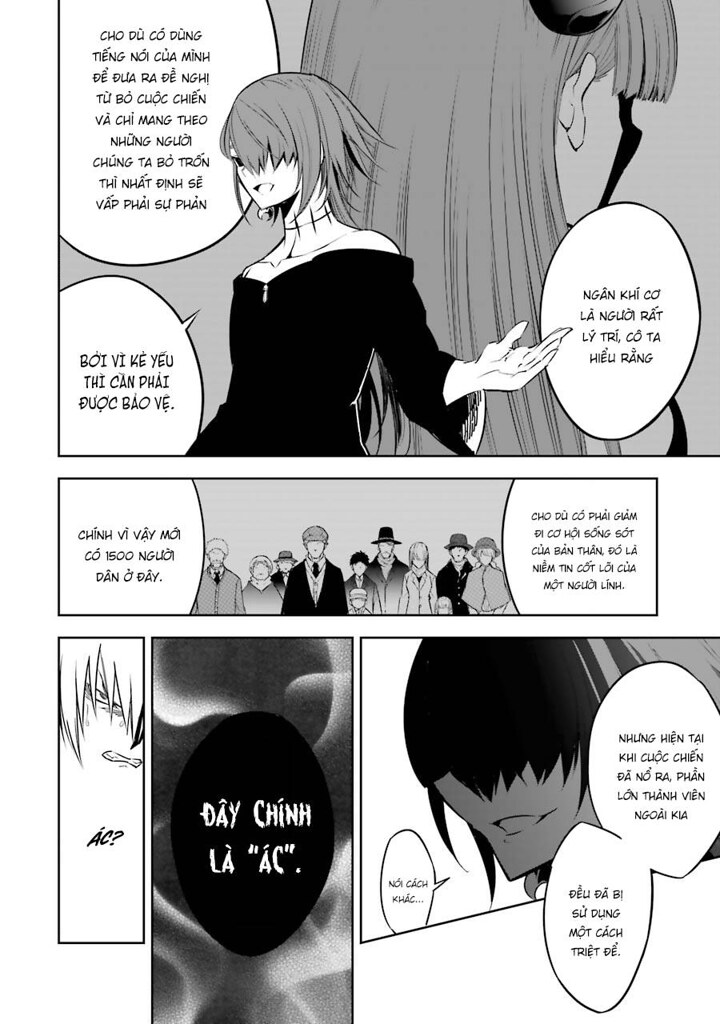This black and white manga frame, illustrated in a portrait orientation, is divided into five distinct panels with Vietnamese text throughout. Dominating the top half of the page, the largest panel features an androgynous character, likely female, with short hair in the front and longer, spiky hair in the back. She is depicted wearing a long black dress that exposes her shoulders. The background includes another female figure with long hair facing away. Surrounding this character are multiple text boxes with Vietnamese script, two to her left and one to her right, which she appears to be pointing toward.

Beneath this, in the center of the page, lies a horizontal strip showcasing a crowd of people facing the viewer. Partial text boxes with Vietnamese characters flank this crowd on either side. 

The bottom third of the page is split into three smaller panels. The left panel presents a boy's face with surrounding speech bubbles, the middle panel contains a black oval with white Vietnamese text, and the right panel features another male character with three text boxes around his head. The entire composition exemplifies traditional manga style, carefully balancing detailed character illustrations with rich conversational content.